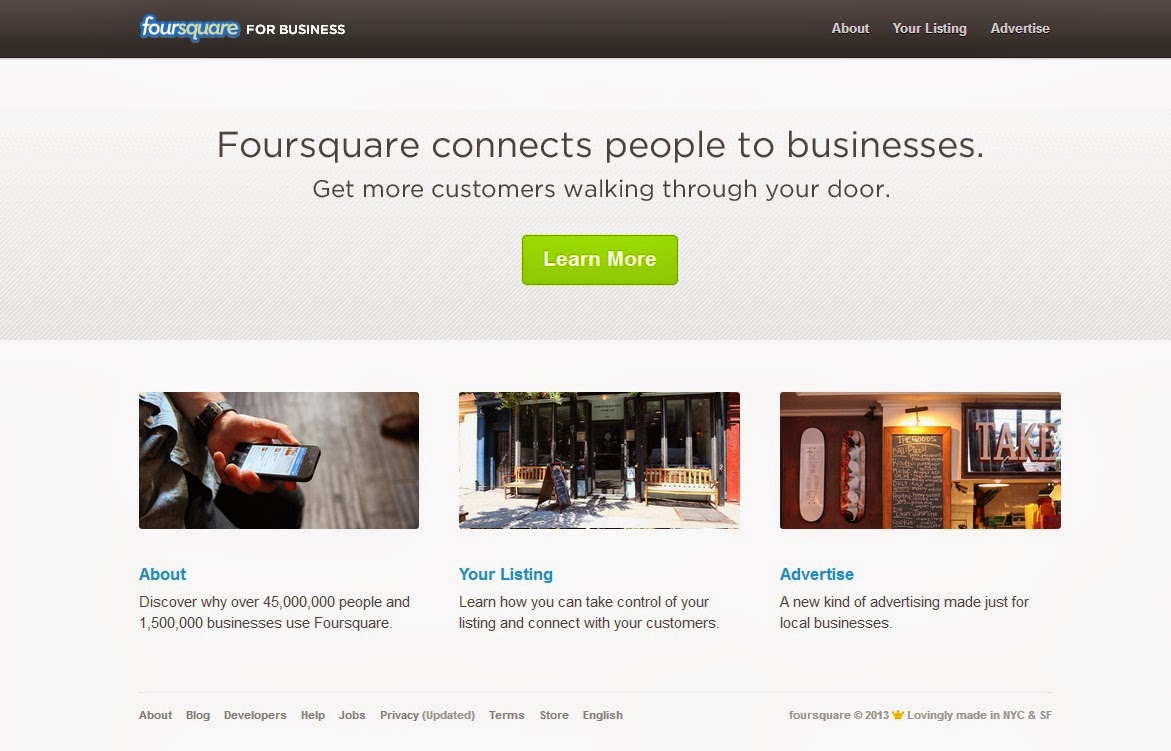This landscape-oriented image captures a detailed view of a Foursquare website page. At the top, a thin, black rectangular border features the Foursquare logo, a light blue outline enclosing a white interior. Adjacent to the logo, the phrase "For Business" is displayed in white. To the right, additional clickable options read "About Your Listing" and "Advertising" in white text. Below this section, a gray box with black lettering proclaims, "Foursquare connects people to businesses. Get more customers walking through your door." Inside the gray box, a prominent green button with white text invites users to "Learn More."

A slightly lighter gray box follows beneath, larger in size and containing three images, each accompanied by informative text. To the left, the first image shows a left hand holding a cellphone, captioned with, "Discover why over 45 million people and 1.5 million businesses use Foursquare." The central image depicts a storefront with a message that encourages users to "Learn to take control about your listing and connect with your customers." The final image to the right illustrates the interior of a store with a chalkboard, emphasizing a new kind of advertising tailored for local businesses with the caption, "Advertise. A new kind of advertising made for local businesses."

At the very bottom of the photo, navigation options are available to help scroll through the website seamlessly.